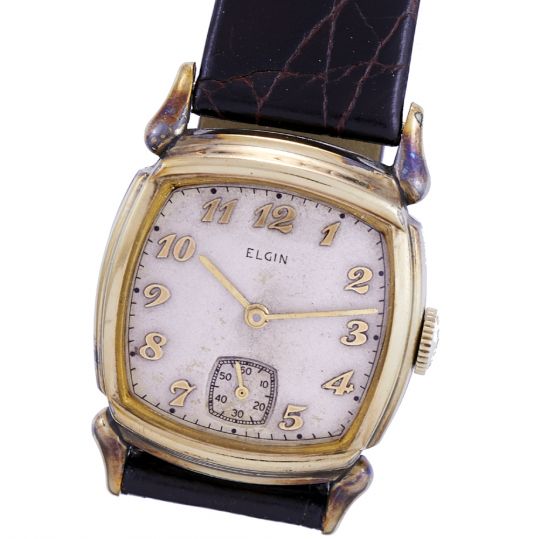The photograph showcases an old Elgin watch positioned at a diagonal angle against a plain white background. The watch face is square-shaped with rounded edges, featuring a gold trim that is slightly discolored near the clamps attaching the strap, transitioning from gold to a darker brown or blackish hue. The watch face itself is white, displaying gold numbers from 1 to 12 around the dial, which is centrally placed alongside the gold Elgin logo. The minute and hour hands are also gold, while a smaller sub-dial at the bottom, marked in black numerals from 10 to 60, serves to count the seconds. Part of the aged black leather strap is visible at the top and bottom of the image. The winding button, also gold, is situated on the right side of the watch face. Overall, the focus is on the intricately detailed and slightly aged watch face with its complementary black and gold color scheme.